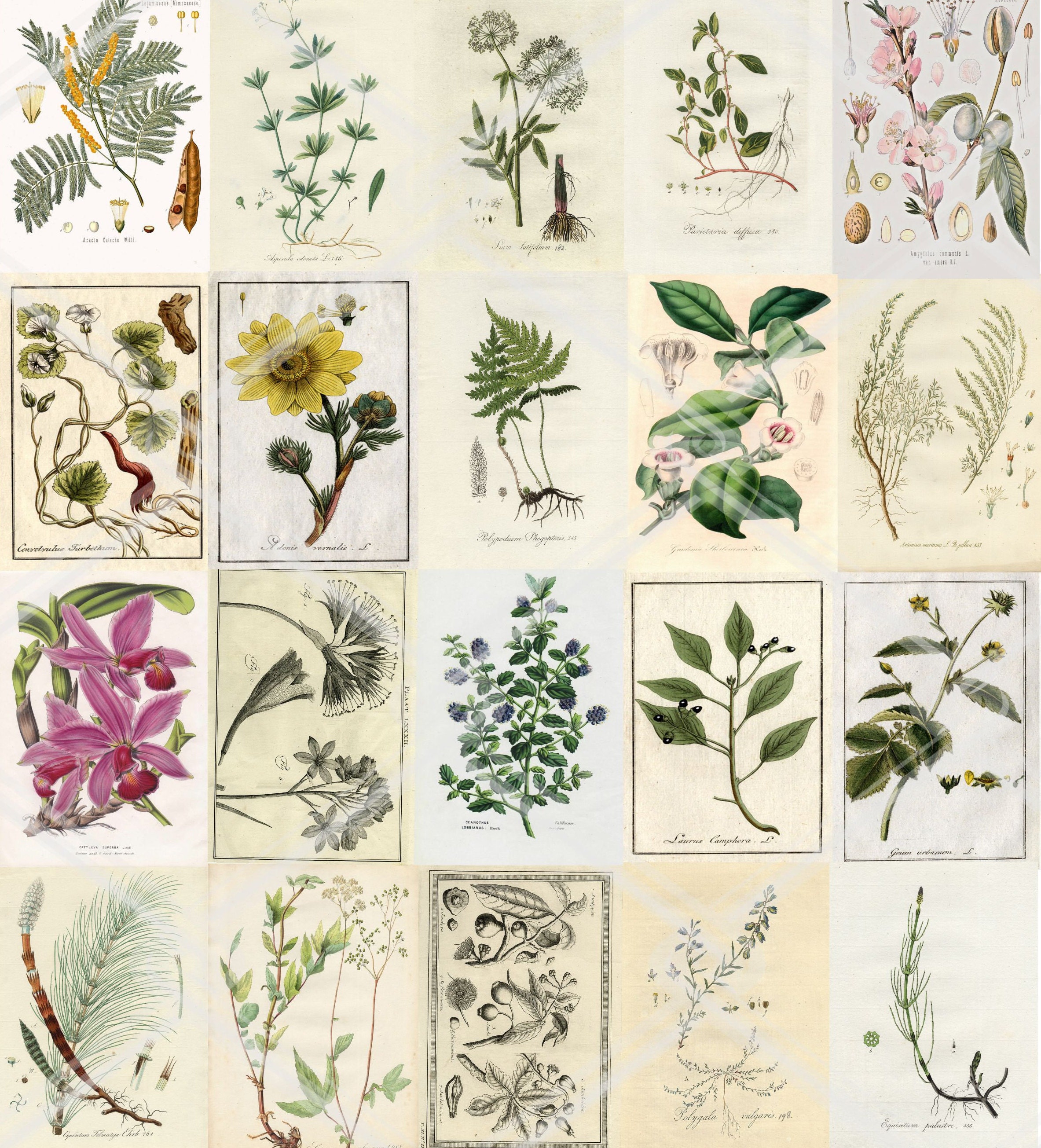The image is a detailed mosaic comprised of 20 botanical illustrations, arranged in a grid with five columns and four rows. Each illustration, roughly the size of a sheet of paper, showcases a different plant with meticulous attention to various aspects, such as foliage, leaf patterns, flowers, and root structures. The depictions vary from singular representations to more intricate panels illustrating seed pods, germination processes, and stages of plant development. The backgrounds of the panels range from white to a yellowish hue, and all the illustrations are in color. Notably, each panel includes the name of the plant, often accompanied by its scientific name, suggesting that these illustrations are intended for classification or identification purposes, possibly excerpts from a botanical reference book. Specific details include white bell-shaped flowers in the fourth panel of the second row, five pink-petaled flowers in the first panel of the third row, and a yellow flower in the second panel of the second row. Overall, the collection provides a comprehensive visual guide to plant identification, capturing the diversity and complexity of various botanical species.